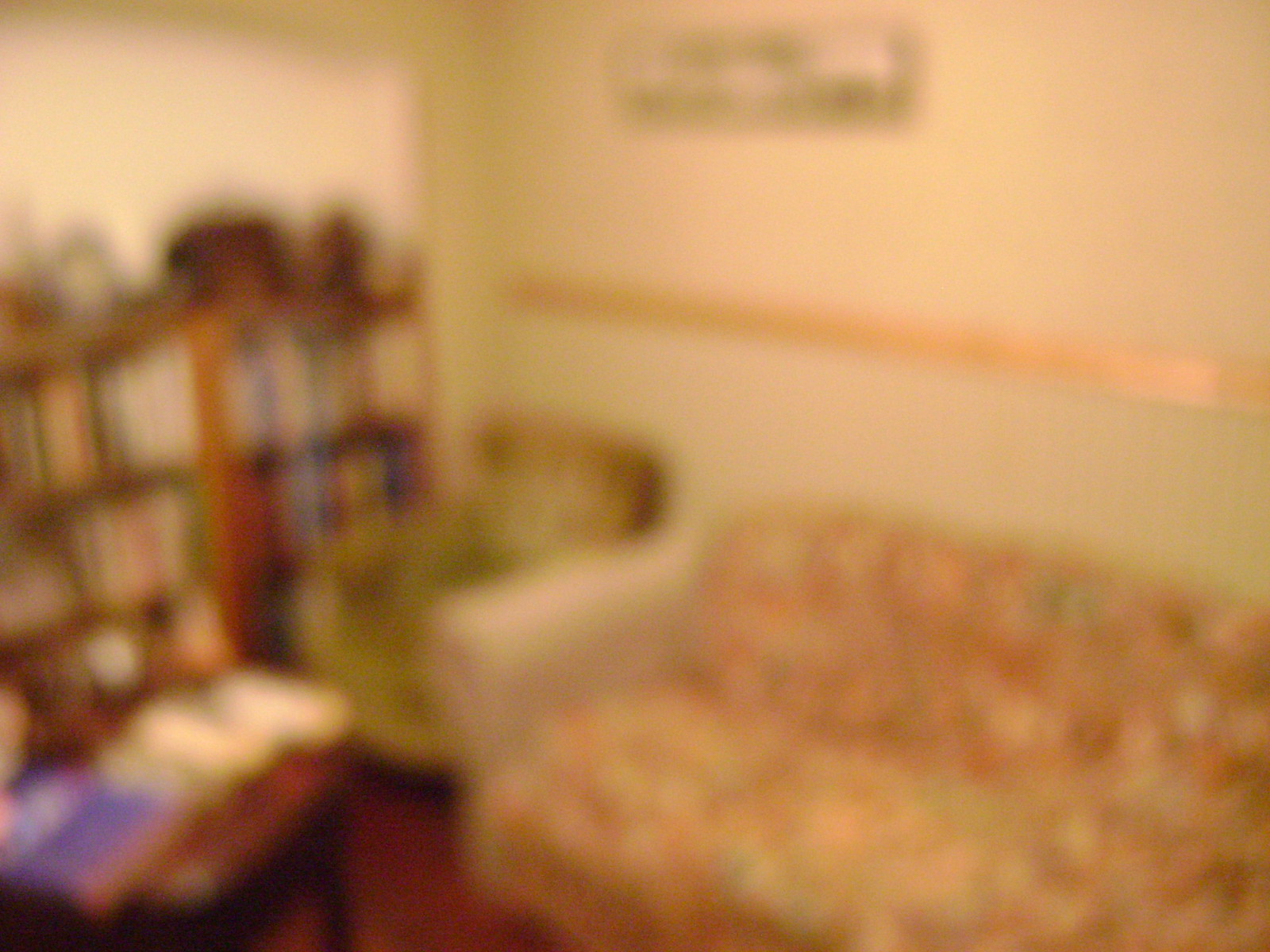This very blurry photograph captures the interior of a cozy reading room or den. The image, taken in landscape orientation, reveals the corner of the room where two walls meet. To the left is a neon lime green wall with a white, whiteboard-like feature on top, and to the right, a lighter green wall. Dominating the scene are two large wooden bookshelves, filled with vertically arranged books of various colors including blue, red, white, and green. In front of the left bookshelf, there is a floral couch, which appears orangey-red and has a cream-colored armrest. One of the shelves features brown, boxy decorations alongside what appears to be a statue. Adjacent to the couch, nestled in the corner, is a pea green armchair. Above this chair hangs a framed picture. Sitting in front of the couch is a dark wooden coffee table, adorned with an assortment of books, including a noticeable purple one. The room has a rust-colored carpet and halfway up the walls is white-painted paneling, topped by a peachy pink border, with the remainder of the wall up to the ceiling being white plaster. The details, though blurry, give a warm and cluttered character to this intimate living space.